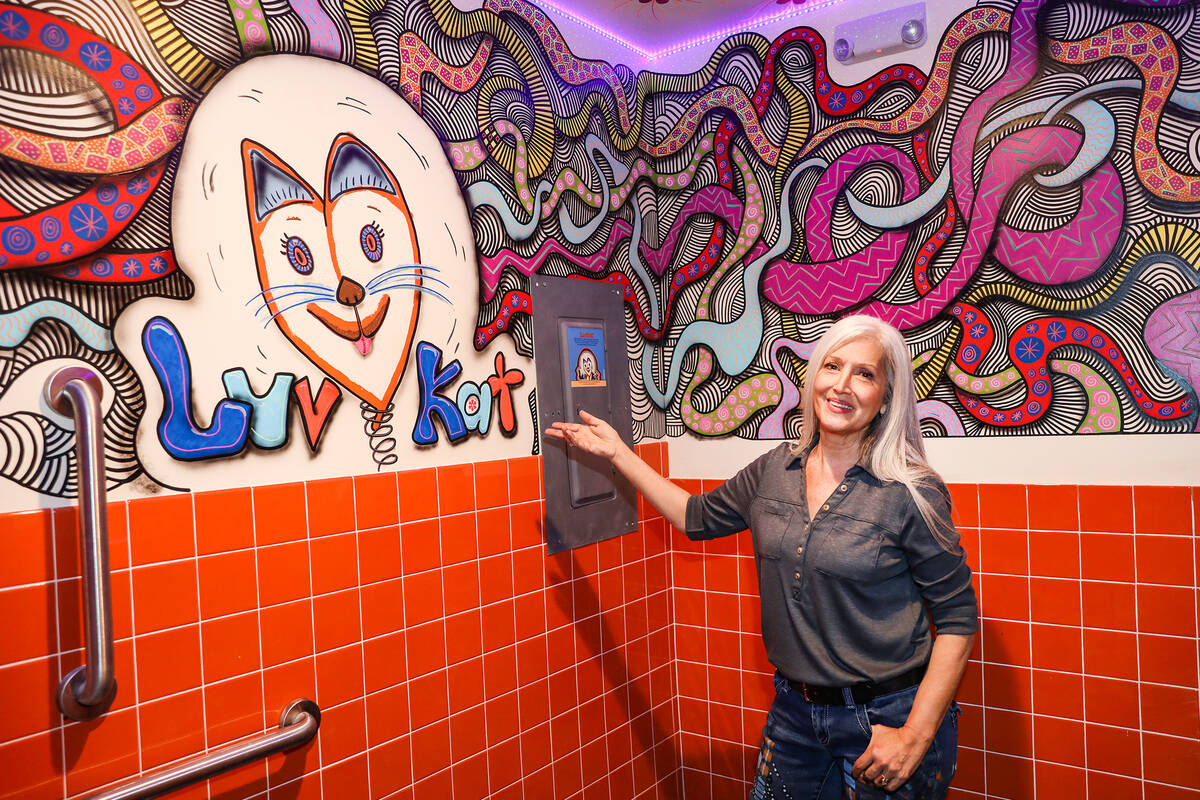In this vibrant and artistic bathroom, the focal point is an older, tan Caucasian woman with flowing silver hair, wearing a dark-colored top, possibly a black or dark red long-sleeve button-down shirt. She appears to be smiling broadly, her head tilted slightly to the right, giving off a warm and inviting aura. The bathroom walls are a canvas of creativity, adorned with gray-striped, snake-like patterns intertwining across a red tile backsplash. Prominently featured in the mural is the phrase "Love Cat" amidst whimsical and dynamic designs. This bathroom, with its unique and artistic decor, offers an intriguing and photo-worthy backdrop, capturing the woman in an environment that blends sophistication and playful artistry.